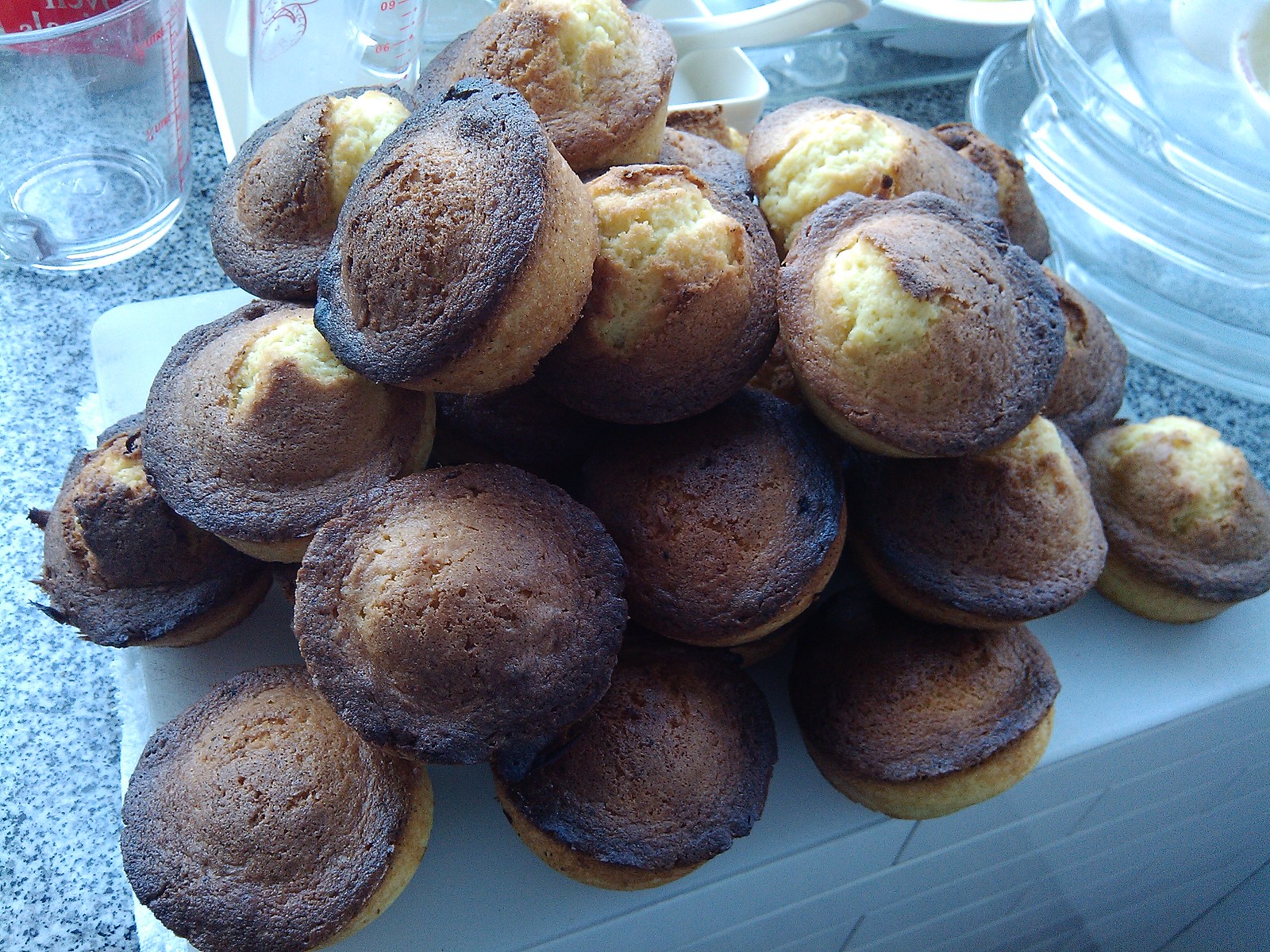This photograph captures a heap of muffins, artfully stacked in a nearly triangular pyramid shape, resting on a kitchen countertop that appears to be made of stone, possibly marble or granite. The muffins, approximately twenty in number, display a golden yellow cake through their cracked tops, surrounded by darker, slightly overcooked edges. Each muffin has a heaped, rounded top, enhancing their rustic appearance. The scene is set in a well-used kitchen area, with measuring jugs, transparent glass Pyrex dishes, and ceramic trays visible in the background, adding depth and context to the image.